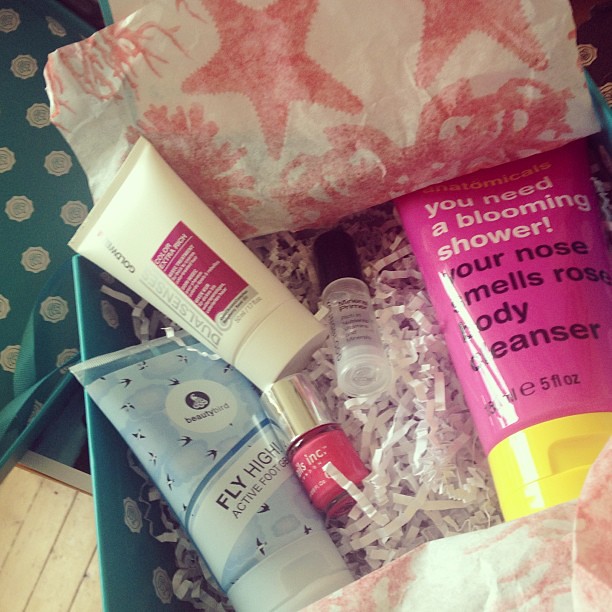The image depicts an open turquoise gift box adorned with small, indistinct icons on its exterior. Inside, the box is filled with crinkled, confetti-cut designer packing paper. Within the box are several beauty products: a turquoise tube labeled "Beauty Bird Fly High Active Foot Gel," a pink tube with a yellow cap labeled "Anatomicals: You Need a Blooming Shower? Your Nose Smells Rose Body Cleanser," a white bottle with a pink box that is partially blurred and indecipherable, and a translucent spray bottle that is also blurry and unreadable. There is a jar of dark pink nail polish marked with "INC" in white text. The overall presentation is colorful and thoughtfully arranged, with each product neatly nested among the packing material.